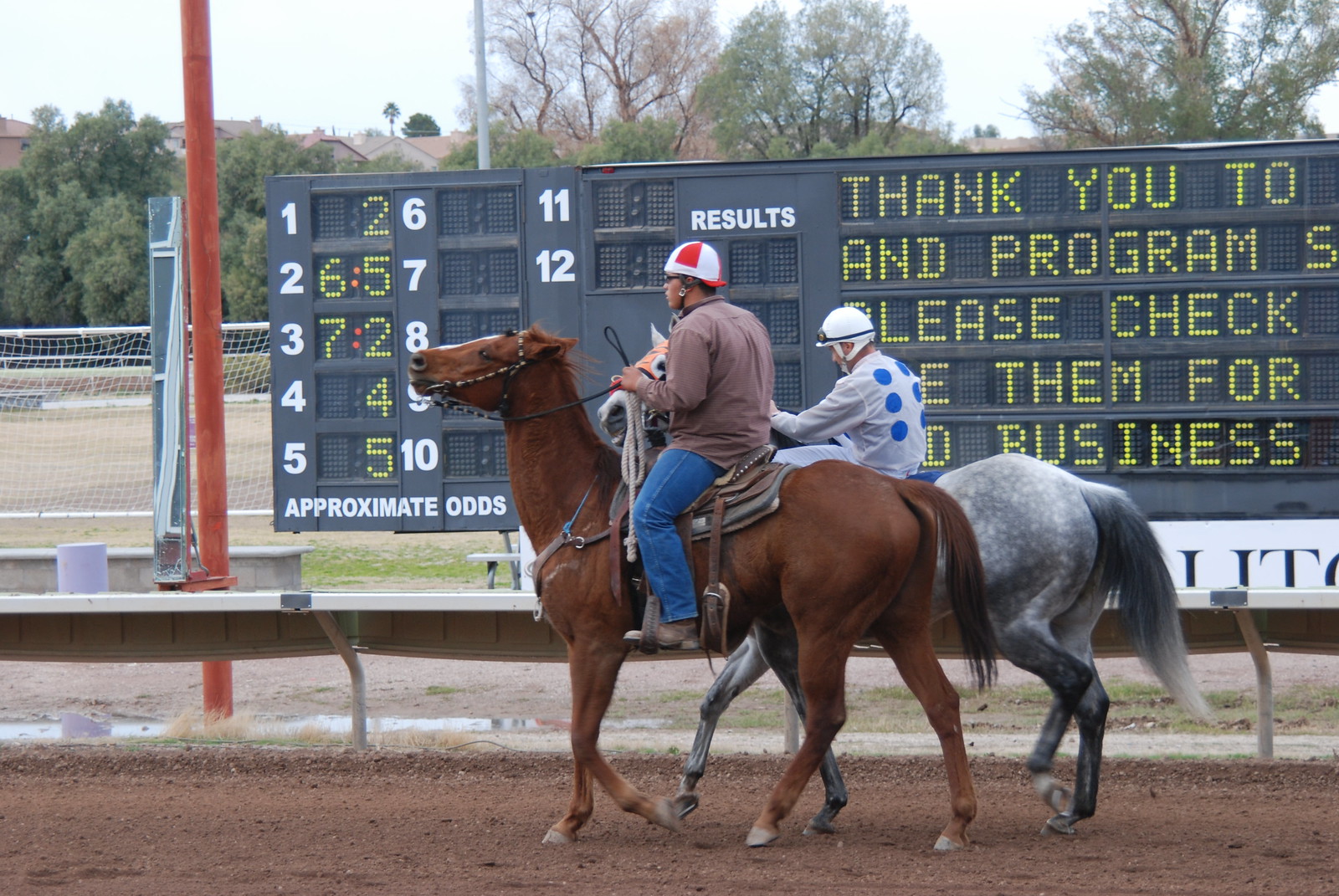The image depicts two horse jockeys riding on a dirt racing track. In the forefront, a Black man is mounted on a brown horse with a white spot on its face. The horse is equipped with a gray saddle blanket and a light brown saddle. The jockey is wearing a long-sleeved brown shirt, blue jeans, and brown boots, and on his head, he has a red-and-white striped jockey helmet secured with a black strap. Riding slightly behind, another jockey is partially obscured but visible enough to see he has a white shirt with blue polka dots on the back and a white helmet with goggles and a strap. His mount is a gray horse with white spots. 

In the background, the setting includes a grayish-black scoreboard displaying numbers 1 through 12 in white and various odds, with text like "thank you to" and "program, please check." Further back, there's a guardrail, a red pole, and numerous trees lining the horizon. The area around the track features some grass and a hill, adding natural scenery to the sports setting.